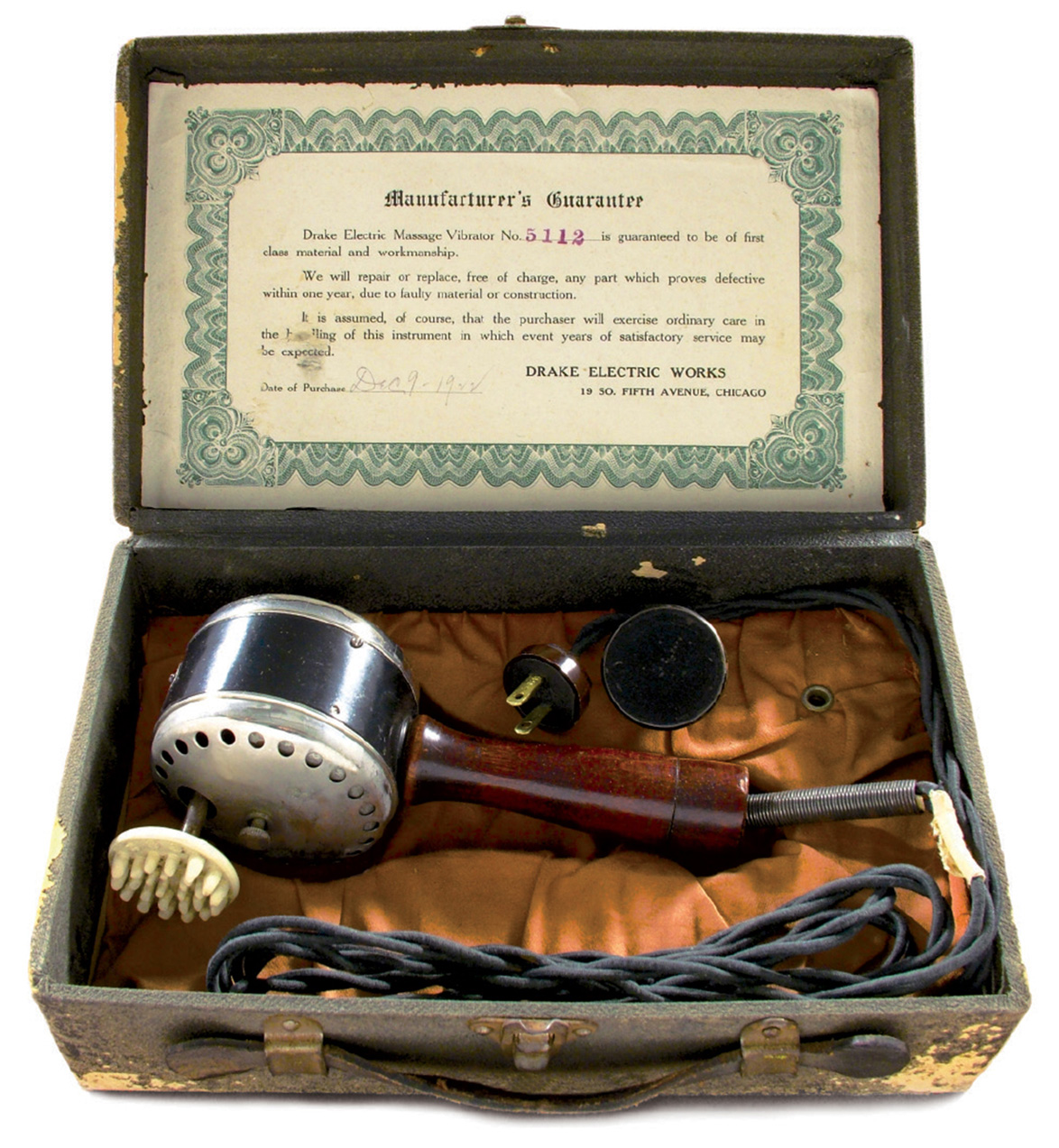This color landscape photograph captures an antique handheld device presented within a worn and aged box that bears the appearance of a decaying, yellowed leather suitcase from a long time ago. The interior of the box features an upper lid lined with a cream-colored certificate bordered in dark green. The certificate, issued by Drake Electric Works, is titled "Manufacturer's Guarantee" and provides details guaranteeing the device dated December 9, 1902. The lower part of the box is lined with a mustard-brown cloth, upon which rests the antique device. This device, identified as a Drake Electric Massage Vibrator, model number 5112, consists of a wooden handle with a black electrical cord extending from it, indicating it plugs into a wall socket. The handle supports a cylindrical section that leads to a metal piece with a white, spiked attachment, resembling a brush or massage head. The detailed craftsmanship and historical elements give the photograph a sense of photographic representational realism.